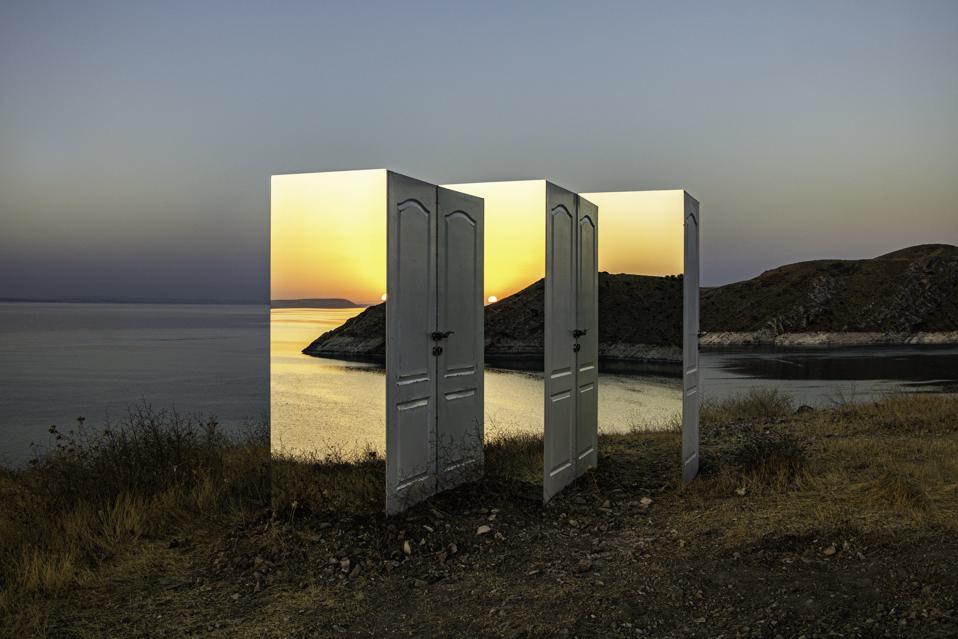The image depicts a surreal, manipulated scene set in a marshy area with a calm, blue body of water. In the background, a distant mountain rises above the far shore. The foreground is marked by dead, brown grass and dirt, evoking a natural yet rugged terrain. In the center of this landscape stand three large, chrome-like rectangular boxes, each featuring two white doors with handles. These doors are ajar, presenting a surreal contrast: while the image outside the doors is dimly lit, likely at dusk or dawn with warmer hues, the scene viewed through the doors is noticeably different. Inside the doors, the landscape appears as though illuminated by a vivid sunrise or sunset, enhancing the illusion. The water remains undisturbed, reflecting the distorted yet captivating blend of reality and illusion. The juxtaposition of these brightly lit, picturesque glimpses against the more muted, natural surroundings creates a striking, almost dream-like composition.